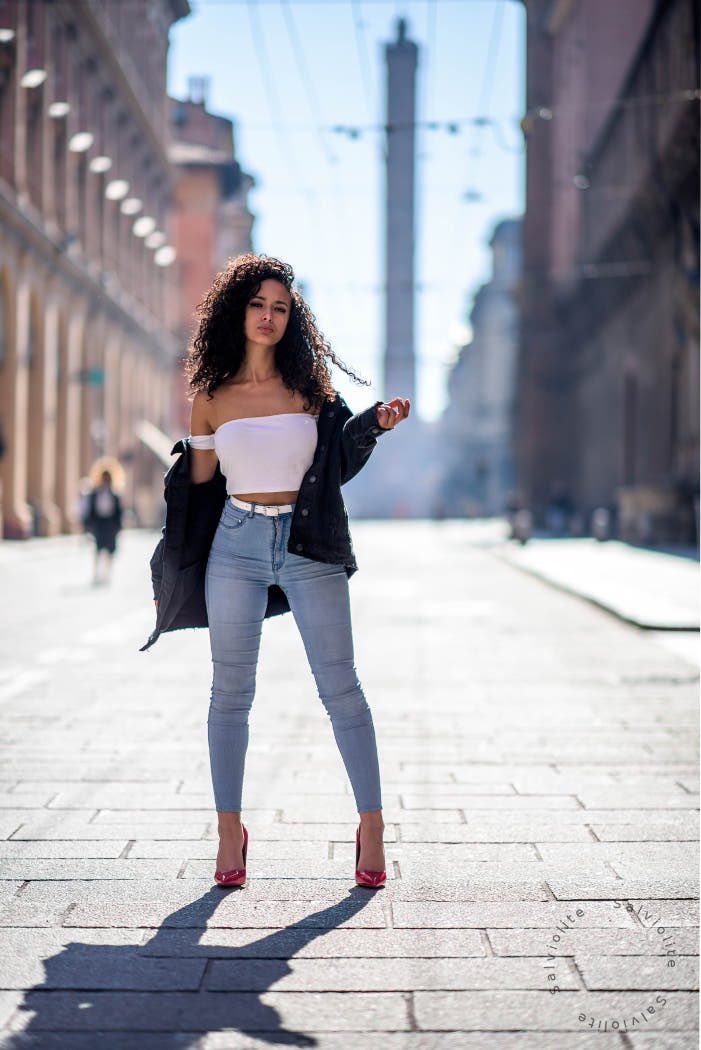In the image, a young woman with an olive skin tone stands confidently in the middle of a cobblestone street, posing for the camera. She wears striking red high-heel shoes and tight-fitting blue jeans cinched with a white belt, which accentuate her legs. A cropped, sleeveless white top reveals her midriff, while a black jacket hangs loosely off her right shoulder. Her long, thick, curly dark brown hair cascades down her back. Her left arm is raised, with fingers pointing forward, and she appears to be holding a lock of her hair. The background features out-of-focus tall, 1800-style buildings, hinting at a European cityscape, with a noticeable tower rising up behind her left side.